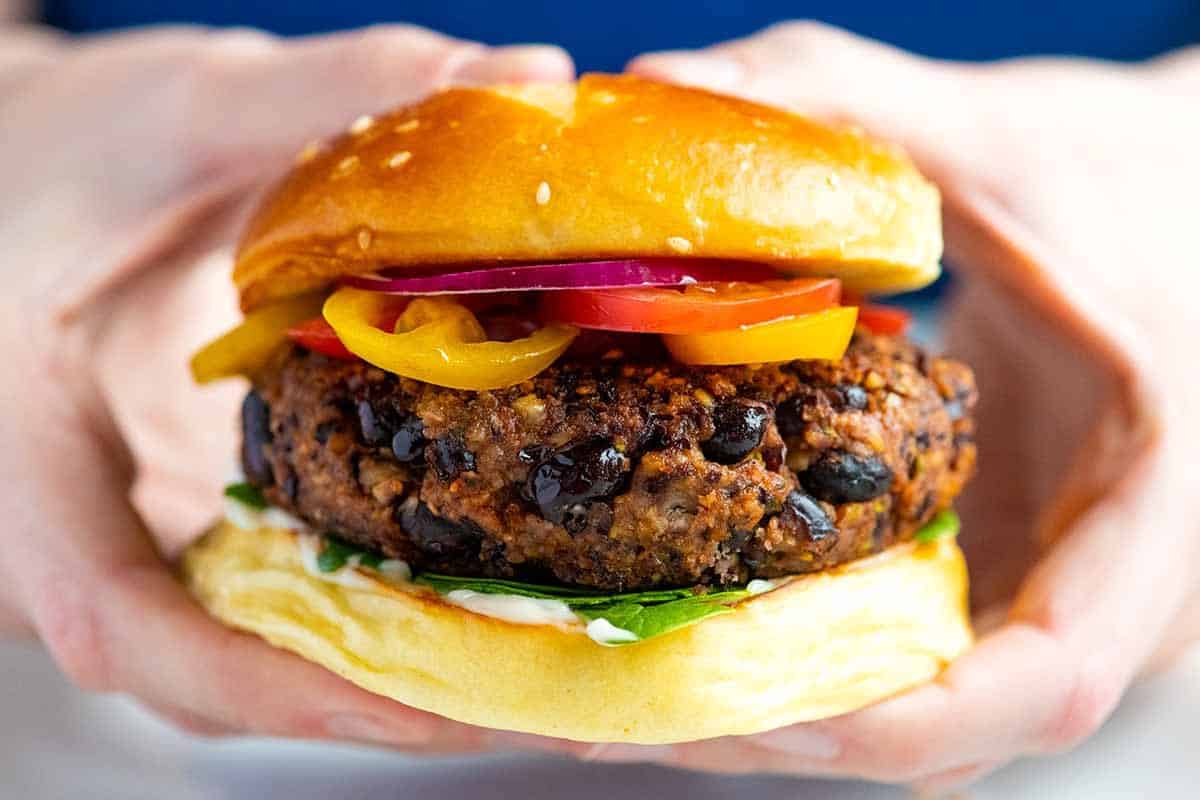In this image, a Caucasian person is holding a black bean veggie burger with both hands, framed against a blue-and-white background. The burger is on a sesame seed bun, golden on top and flatter on the bottom, and it’s bursting with colorful ingredients. You can see black beans and possibly some quinoa or corn mixed into the patty. Garnishing the burger are vibrant slices of red tomato, yellow pepper, pink red onion, and spinach. The base of the burger also features a generous layer of mayonnaise. The carrier of the burger, dressed in a blue shirt and probably khaki pants, presents the burger held with their thumbs on the top bun and their fingers supporting the bottom, against a clean backdrop.